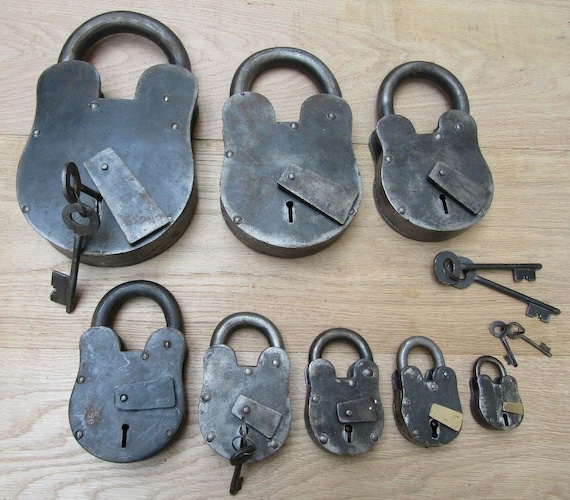The photograph showcases a flat lay arrangement of several vintage metal padlocks and keys on a light tan wooden surface with dark wood grain patterns. The locks, dating from the late 18th century to the early 20th century, are meticulously placed in two horizontal rows. The top row features three large, dark gray metal locks, the largest situated in the upper left corner with a key inserted into its locking mechanism. Adjacent to it are two slightly smaller locks, each characterized by rounded metal openings at the top and exposed keyholes. Below this trio, two vintage 18th-century style keys rest. The second row beneath consists of five increasingly smaller, distressed, and worn locks, arranged from left to right. Again, at the far right of the bottom row, two more vintage-style keys lie just above the smallest lock. The overall composition emphasizes the progression in size and age of these historical locks and keys.